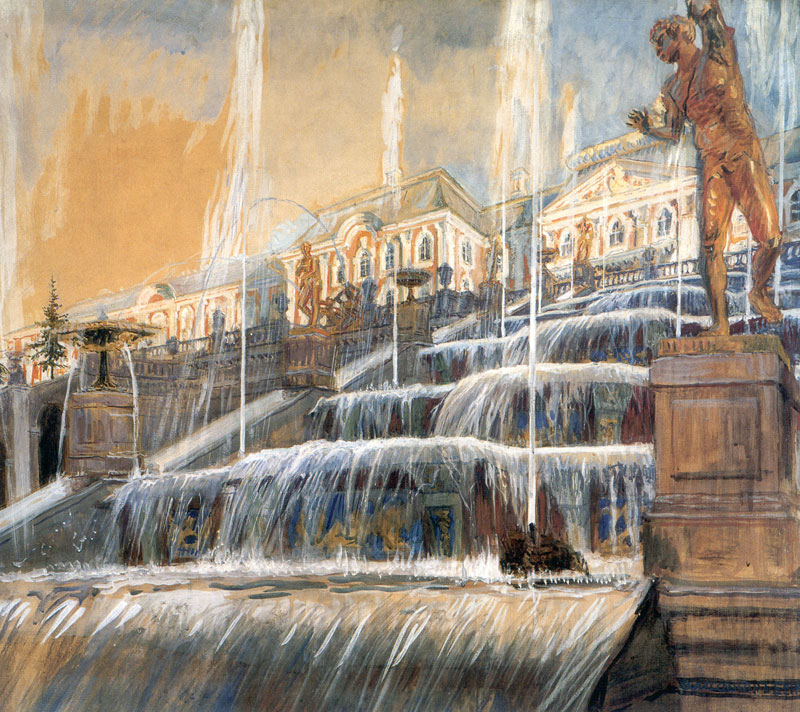The image depicts a grand and intricate scene dominated by a sprawling art installation of cascading waterfalls, each a level higher than the last, creating a dramatic and multi-tiered effect. The waterfalls, adorned with grayish and white water, tumble over one another in a mesmerizing display. To the right of the image, perched on a tall column, is a striking bronze statue of a man, arm raised as if surveying the scene. This statue imparts a historical feel to the composition, perhaps reminiscent of ancient times. Across from him, another bronze statue stands in a crouched position, seemingly engaged with the man and the cascading water.

Above this elaborate setup lie buildings with an orange exterior and white-framed arched windows, reminiscent of a grand mansion or estate. These buildings provide a vivid backdrop with their impressive size and detail, suggesting a structure that could house over a hundred rooms. The sky above is a beautiful blend of orange, cream, and blue hues, with partial cloud coverage adding depth and dimension to the scene. The overall atmosphere is one of historical grandeur, where bronze statues and a monumental water installation harmonize under a richly colored sky.